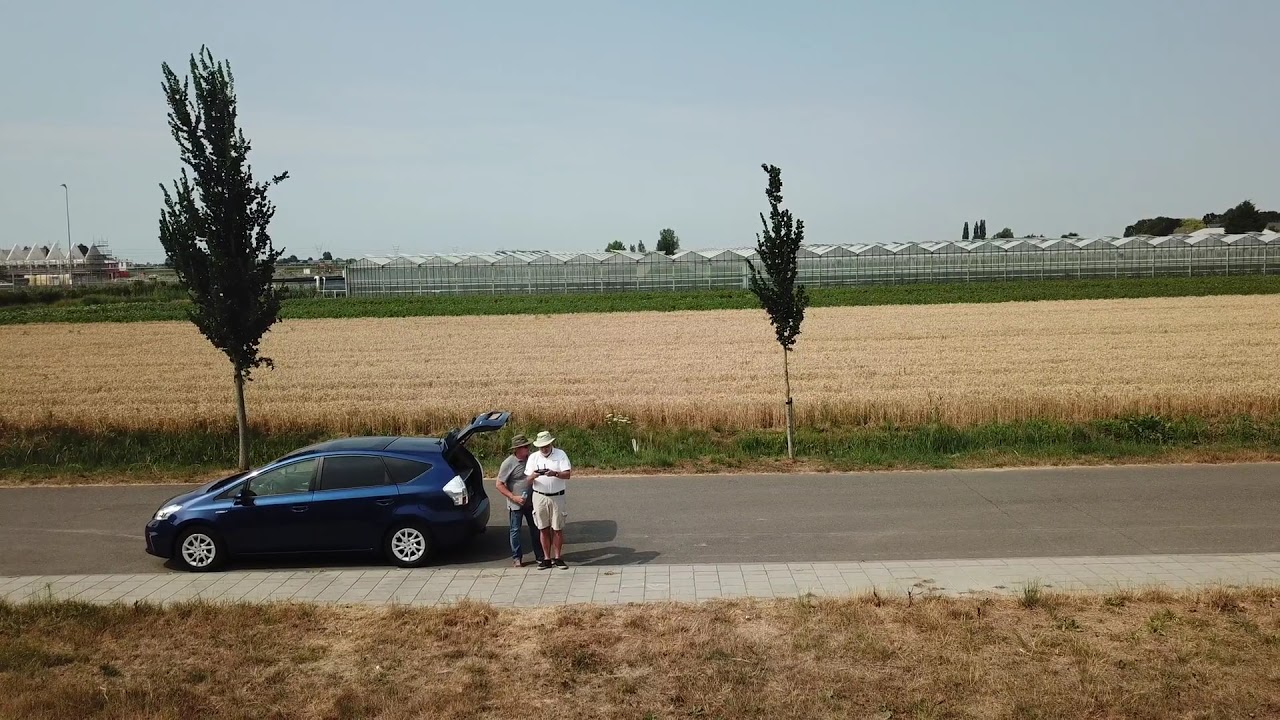In this photograph, we see a tranquil street scene featuring a blue hatchback car parked facing left, with its trunk open. Two men are standing at the rear of the vehicle. One man, dressed in jeans, a gray short-sleeved t-shirt, and a green hat, is next to another man who wears beige shorts, a white short-sleeved shirt, a brown belt, black tennis shoes, and a brimmed hat; he has a white beard. They seem to be engaged with something in the trunk, possibly indicating some roadside situation.

The street is lined with a narrow gray sidewalk and sparse, burnt-looking grass. Across the road, there is a vast expanse of tan, clipped wheat or hay fields. In the background, a row of single-story greenhouses with A-frame roofs stretch neatly along the horizon, enclosed by a protective fence. The setting is likely warm, suggested by the dry grass and the clear, light blue sky without any clouds. Two slender trees punctuate the scene, further enhancing the rural and serene atmosphere.